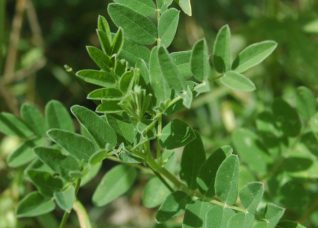This is a close-up, rectangular photograph showcasing a green plant with multiple stems and branches, each adorned with small, narrow, oblong leaves arranged oppositely along the stems. The leaves, which are smooth-edged and slightly fuzzy, are displayed prominently with most pointing upwards and slightly to the left. The image captures the tip of the plant's multiple-leaved branches, each bearing between seven to nine leaves. In the center of the plant, a rosette of new leaves is emerging. The background features a blurred tapestry of various shades of green, brown, and black vegetation, providing a soft contrast to the sharply focused foreground, though it is unclear whether this background consists of the same or different types of plants. The sunlight bathes the plant, highlighting its detailed structure and multiple shades of green with occasional brown accents.